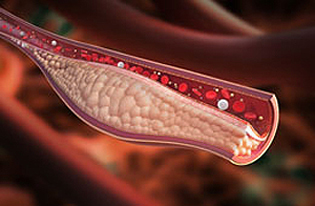The image is a detailed, color illustration of a cross-section view of a vein, depicted in landscape orientation. The vein appears half-open in a tubular, half-circle structure, with the top left being smaller and expanding towards the bottom right, drawing focus to this main vein structure. In the front of the vein, red, white, and blue blood cells are visible, approximately 75 in total, all moving towards the right side of the image. Nestled beneath these blood cells is a prominent, bumpy white pouch with a scaly texture, resembling snake skin. This pouch creates a bulbous bulge in the vein, indicative of a build-up of plaque or cholesterol. The background features faintly visible, blurred repetitive structures, likely more veins or surrounding tissue. The entire scene mimics the scientific aesthetic typical of biology textbooks.